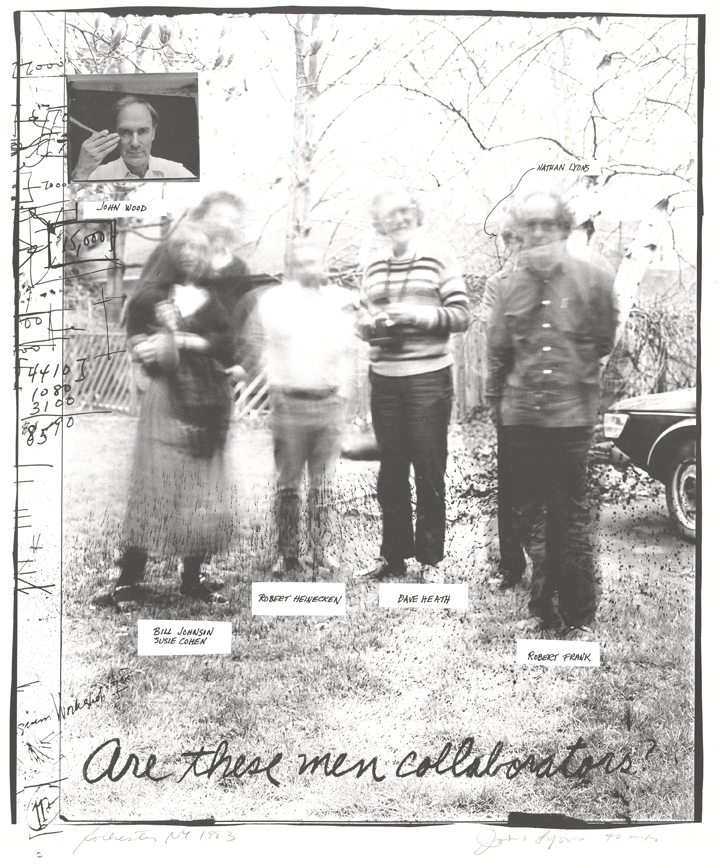The black and white image in question features a blurred group of four older men standing in a semicircle on a lawn, with bare trees and fallen leaves behind them. Each of these men is identified by names inscribed underneath their images at the bottom of the poster: Bill Johnson, Susie Cohen, Robert Heineken, Dave Heath, and Robert Frank, with Nathan Lyons also included. The poster's bottom bears the handwritten script, "Are these men collaborators?" A square in the upper left corner displays a head-and-shoulders portrait of another man, identified as John Wood. To the right, part of a car, specifically a tire and some grass, is visible, adding an additional layer of context to the scene. The overall aesthetic is defined by its monochromatic palette and somewhat chaotic mixture of handwritten notes and numbers scattered throughout the image.